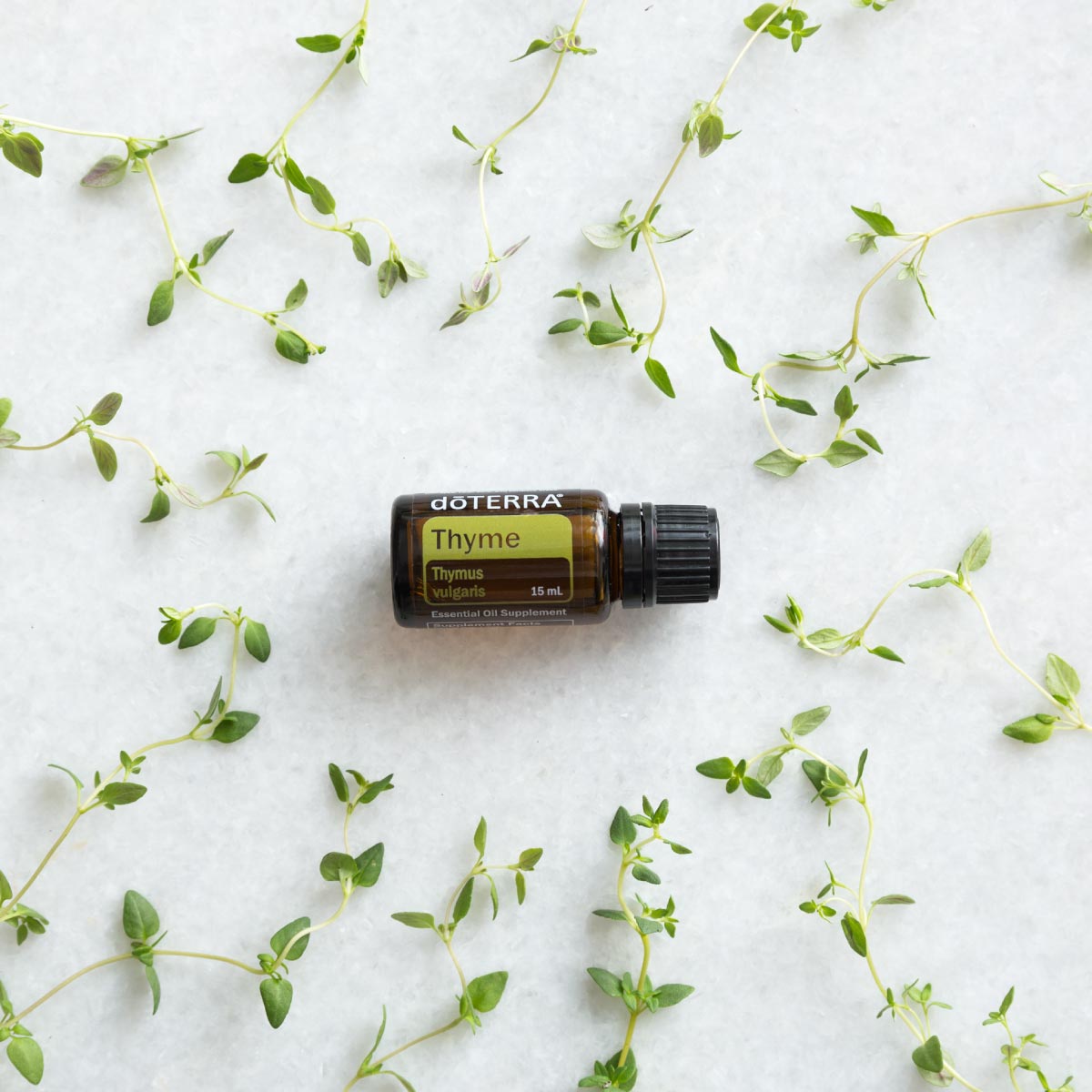This detailed square photograph, approximately six inches by six inches, features a small 15-milliliter bottle of essential oil. The bottle, light brown with a black plastic cap, is positioned at the center of the image, laying on its side with the cap facing right. Surrounding the bottle are delicate, yellowish-green twisting vines adorned with spade-shaped, small green leaves at each bend, creating a circular formation. These tiny leaves are presumed to be from thyme plants. The background of the photograph is a soft, white felt, giving it a fluffy, cotton-like appearance. 

The bottle displays several lines of text in white print. At the top, the brand name "D-O-T-E-R-R-A" is prominently featured, with a distinguishing horizontal line over the 'O'. Below that, on a light green background, the word "THYME" is written. Further down, on a brown background, it reads "THYMUS VULGARIS." Additionally, "Essential Oil Supplement" is printed in white near the bottom of the bottle.